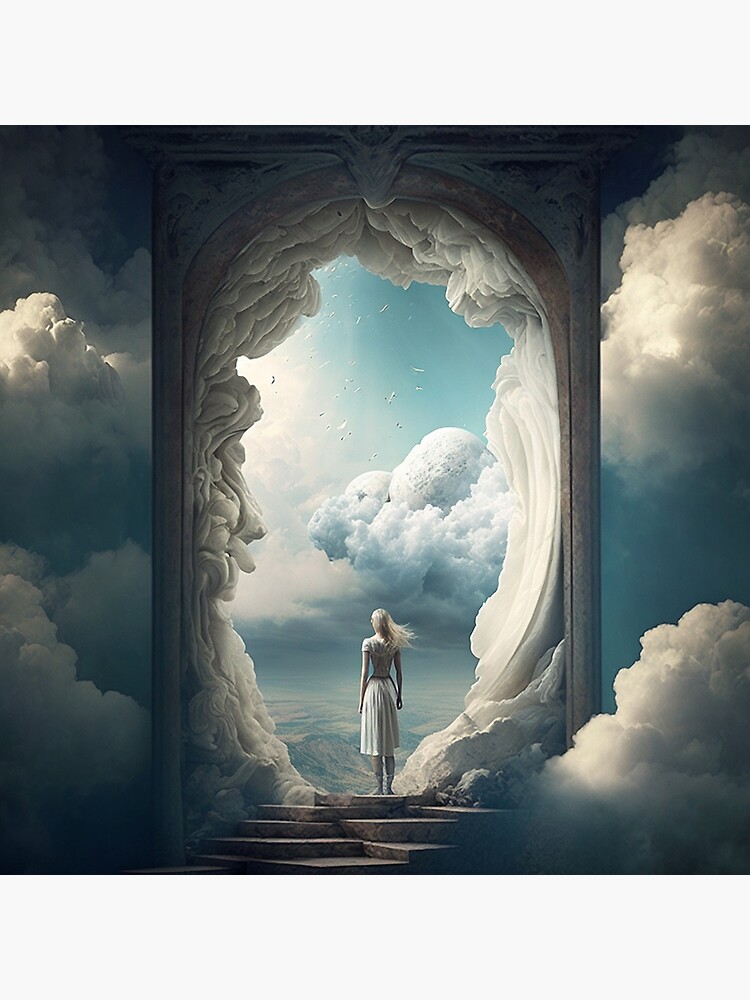A young, slender girl with long, flowing blonde hair stands with her back to us in the center of an oval-shaped archway, reminiscent of a classical Greek or Roman temple. She wears a dreamy whitish-blue dress that falls to her knees. The archway, adorned with decorative clouds, seems to be part of a large, temple-like structure perched high on a mountain, offering a breathtaking and surreal vista. Rolling foothills stretch out below her, blending into a sky filled with big fluffy clouds and the dreamy hues of blue and white. Stone steps lead up to this heavenly-looking threshold, evoking a scene that feels both biblical and otherworldly. The overall palette and composition of the image create an ethereal atmosphere, as if the girl is gazing into the skies of God or a dream-like rendition of heaven.